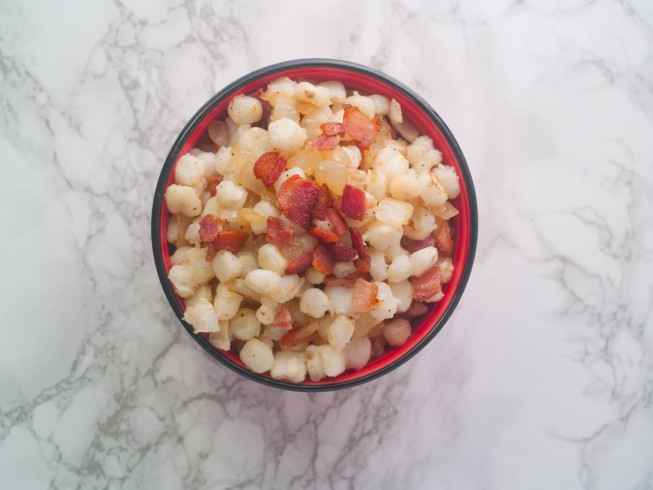In the image, a red-and-black bowl sits on a white and gray marbled countertop, predominantly featuring intricate gray veins on the left side. The bowl, shown from a top-down perspective, has a red interior and a black exterior. Inside the bowl, there appears to be seasoned hominy, resembling small white balls or corn kernels, and it is topped with finely chopped bacon bits scattered across the dish. The detailed countertop and the vibrant bowl contrast each other, creating a visually appealing culinary presentation.